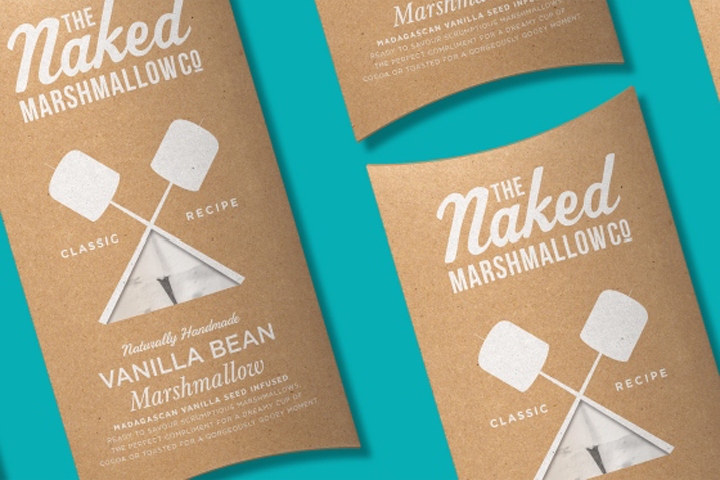The image showcases a meticulously staged product shot of The Naked Marshmallow Company. The primary focus is on the packaging of their Classic Recipe, Naturally Handmade Vanilla Bean Marshmallows, infused with Madagascan vanilla seeds. The rectangular packaging, featuring both curved bottoms on the short sides and curved top and bottom edges, appears to be crafted from a medium brown, unbleached paper that resembles wood. The text is written in white, prominently displaying the brand name and product description. The design includes a teepee-like structure formed by two sticks crossing at the top, each holding large marshmallows. The packaging is angled slightly against a serene turquoise, or seafoam green, background, creating a visually appealing contrast that highlights the product’s artisanal quality. Multiple packages are arranged in the background, further emphasizing the brand's presence in this professional product shot.